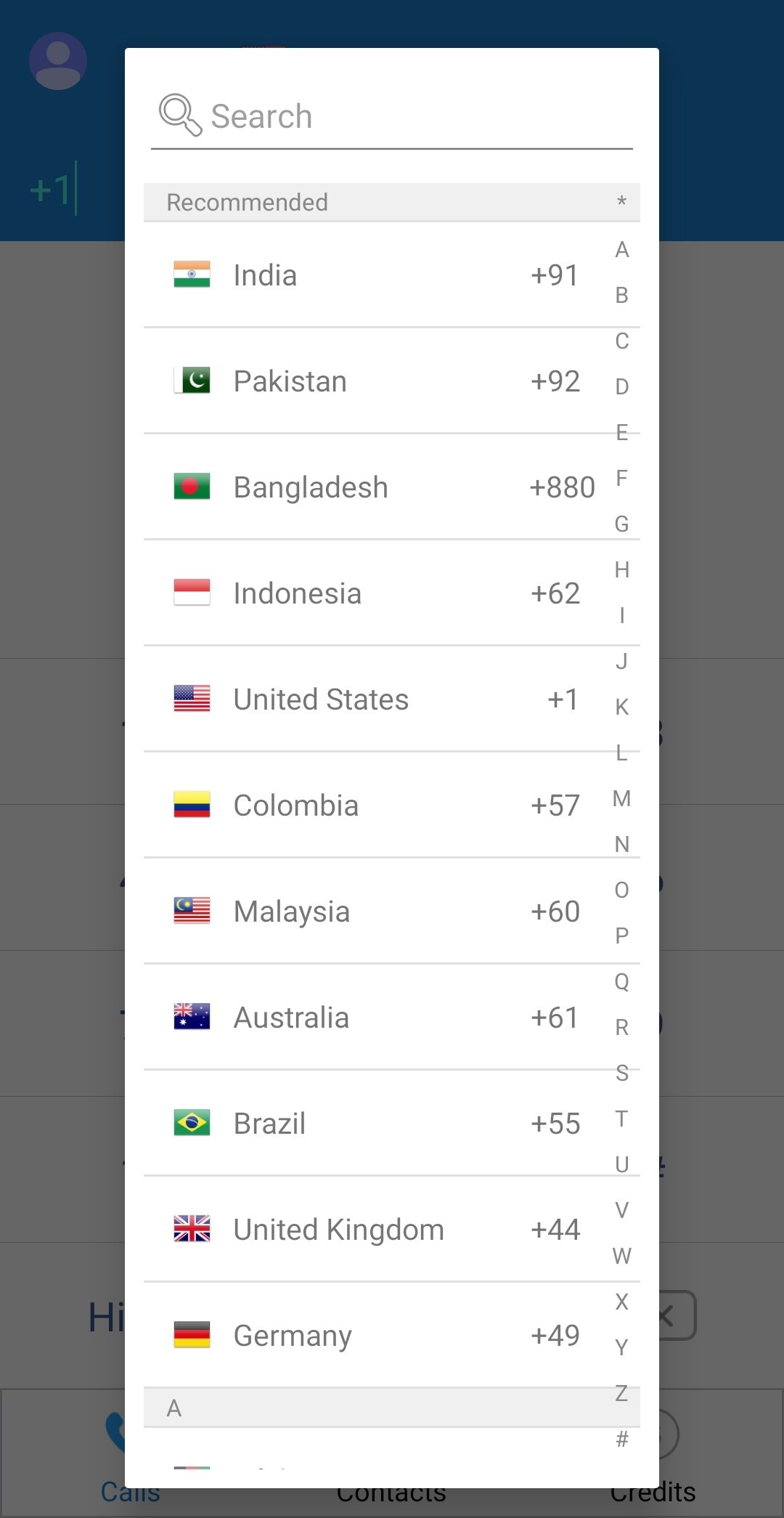The image features a gray background with a prominent, rectangular window superimposed on it. This window has a white backdrop and a vertical orientation. At the top of the window, a "Search" label can be seen alongside a corresponding search bar for user input. Directly beneath this is a "Recommended" heading, under which a list of country names, along with their respective flags, is displayed. Each country entry includes its name followed by its international dialing code, with a line separating each one for clarity.

The detailed list begins with "India +91" at the top, followed by:

- Pakistan +92
- Bangladesh +880
- Indonesia +62
- United States +1
- Colombia +57
- Malaysia +60
- Australia +61
- Brazil +55
- United Kingdom +44
- Germany +49

On the right edge of this window, an alphabetical index from A to Z is arranged vertically, allowing users to quickly navigate through the list of countries.